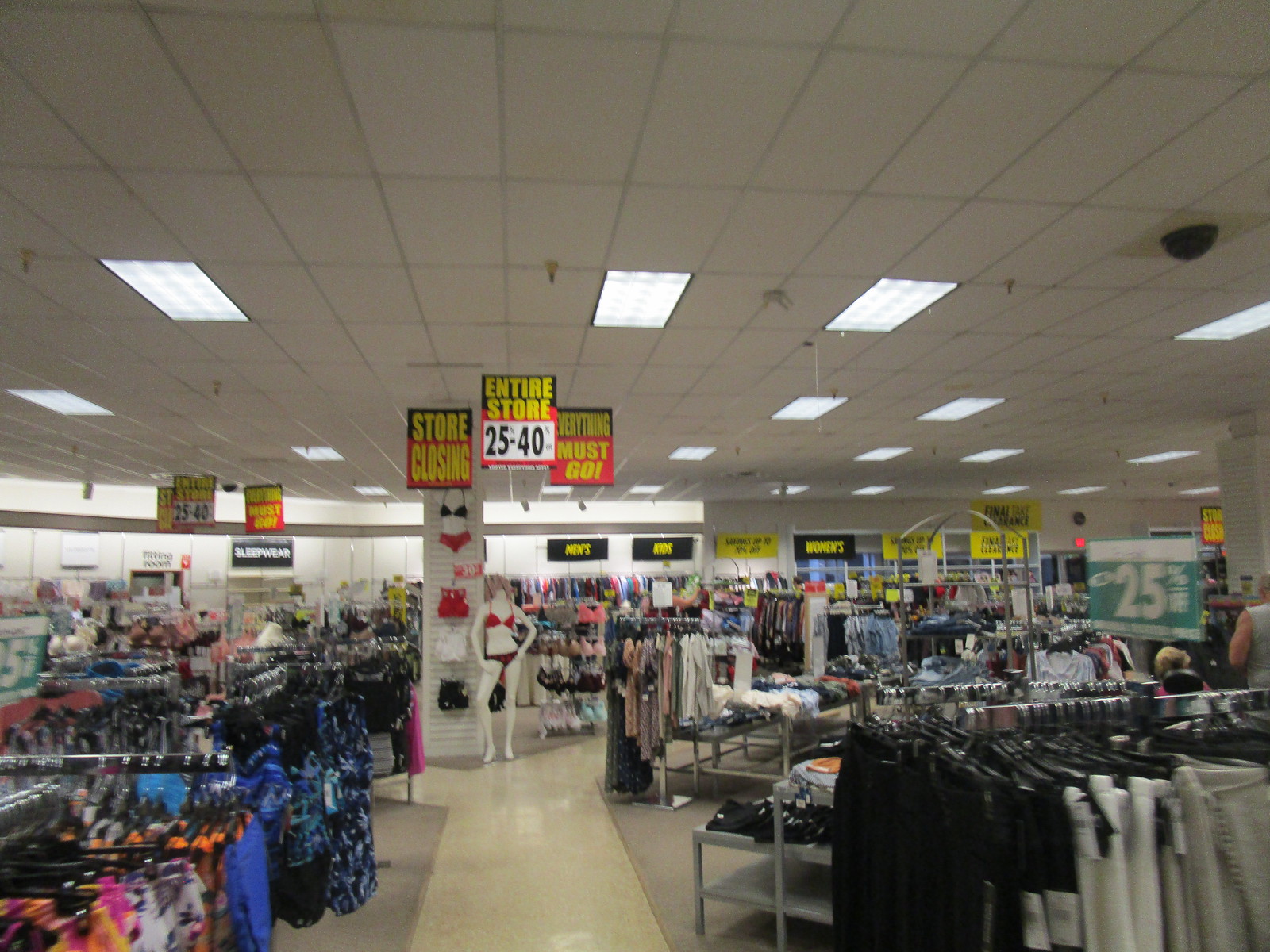The image captures a wide-angle view of the inside of a Sears store that is closing down. Dominating the space are numerous signs hanging from the ceiling, proclaiming "Store Closing" and "Everything Must Go," with discounts ranging from 25 to 40% off. The sale signs feature a distinct color scheme: predominantly black and red, with yellow lettering. The ceiling reveals foam panels held up by metal framework, interspersed with fluorescent lights, and a visible half-dome security camera. Within the store, racks of clothing fill the space, including bathing suits on the left side and various summer outfits on the right. Toward the back, other sections are marked by black signs with contrasting yellow or white writing, indicating areas such as "Sleepwear," "Men’s," and "Kids." Prominently at the end of the center aisle stands a mannequin dressed in a red bikini, under the stark lighting of the retail environment.